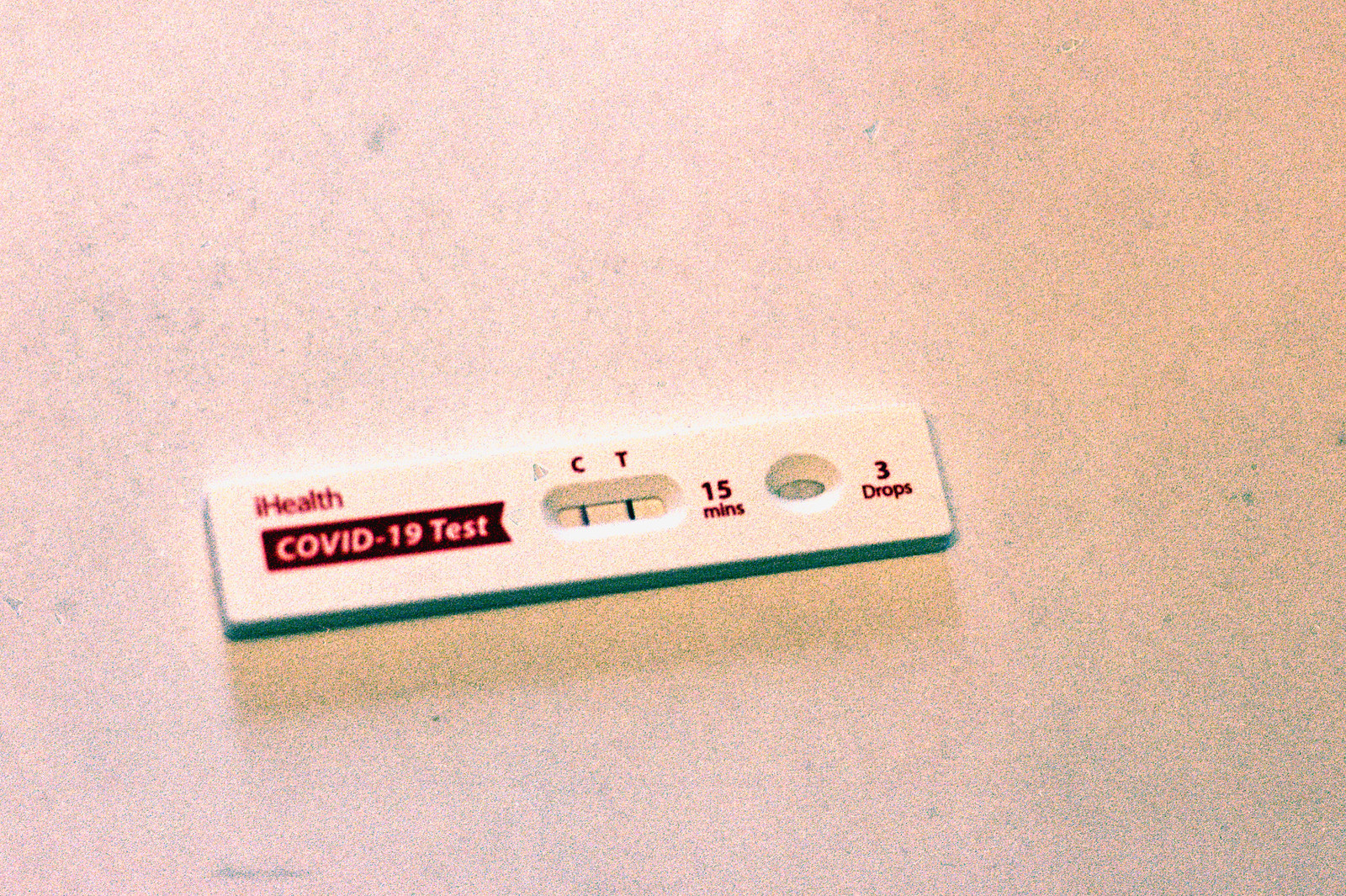This image shows a close-up of a COVID-19 test kit from iHealth. The compact, three-inch rectangular plastic device features the brand name "iHealth" prominently displayed at the top. Just below, a ribbon-like banner clearly reads "COVID-19 Test." Immediately adjacent to this banner is a pill-shaped screen, displaying two horizontal red lines.

Above the screen, the letters "C" and "T" are labeled, indicating the control and test lines of the kit. Further to the side of this pill-shaped area, the instructions "15 minutes" are inscribed, suggesting the waiting time for the test results. To the right, an oval-shaped indent is marked with the instructions "three drops," guiding users on the number of sample drops needed.

The screen and surrounding areas have a pink-red fluorescent hue, emphasizing the test results. The detailed layout ensures ease of use and quick reading of the results within a 15-minute timeframe.